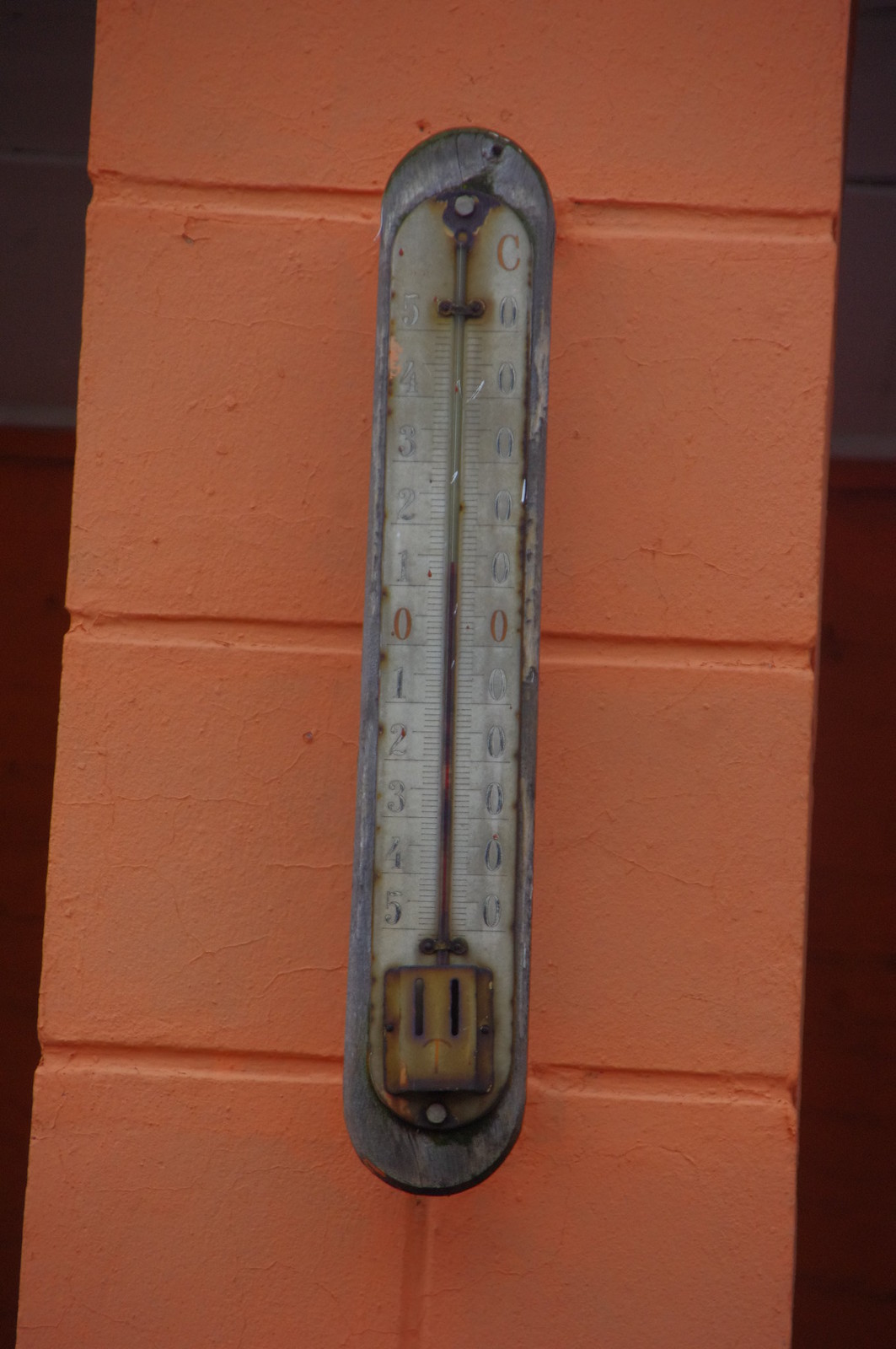This vertical photograph features the edge of an old brick wall, focusing on an aged, metal thermometer. The antique thermometer, made of what appears to be galvanized metal, is the central subject of the image. It is shaped like a long rectangle with rounded ends, reminiscent of looking down on a hot dog. The front surface of the thermometer is flat, displaying a white rectangular area with rounded ends, which is marked with numerical scales.

The thermometer has a red "C" on the upper right side, likely indicating Celsius, and features numbers descending from the top to bottom. The scale is segmented with a red zero in the middle, indicating the midpoint. Above the zero, the numbers decrease from 5 to 1, while below the zero, they increase from 1 to 5. Notably, the other side of the thermometer lacks any additional symbols or markings, suggesting some may have faded or worn off over time.

The center of the thermometer, where the mercury would typically be, is visibly empty, indicating that the mercury is no longer present. The vintage thermometer stands out against the backdrop of the red brick wall, adding character and a sense of history to the scene.